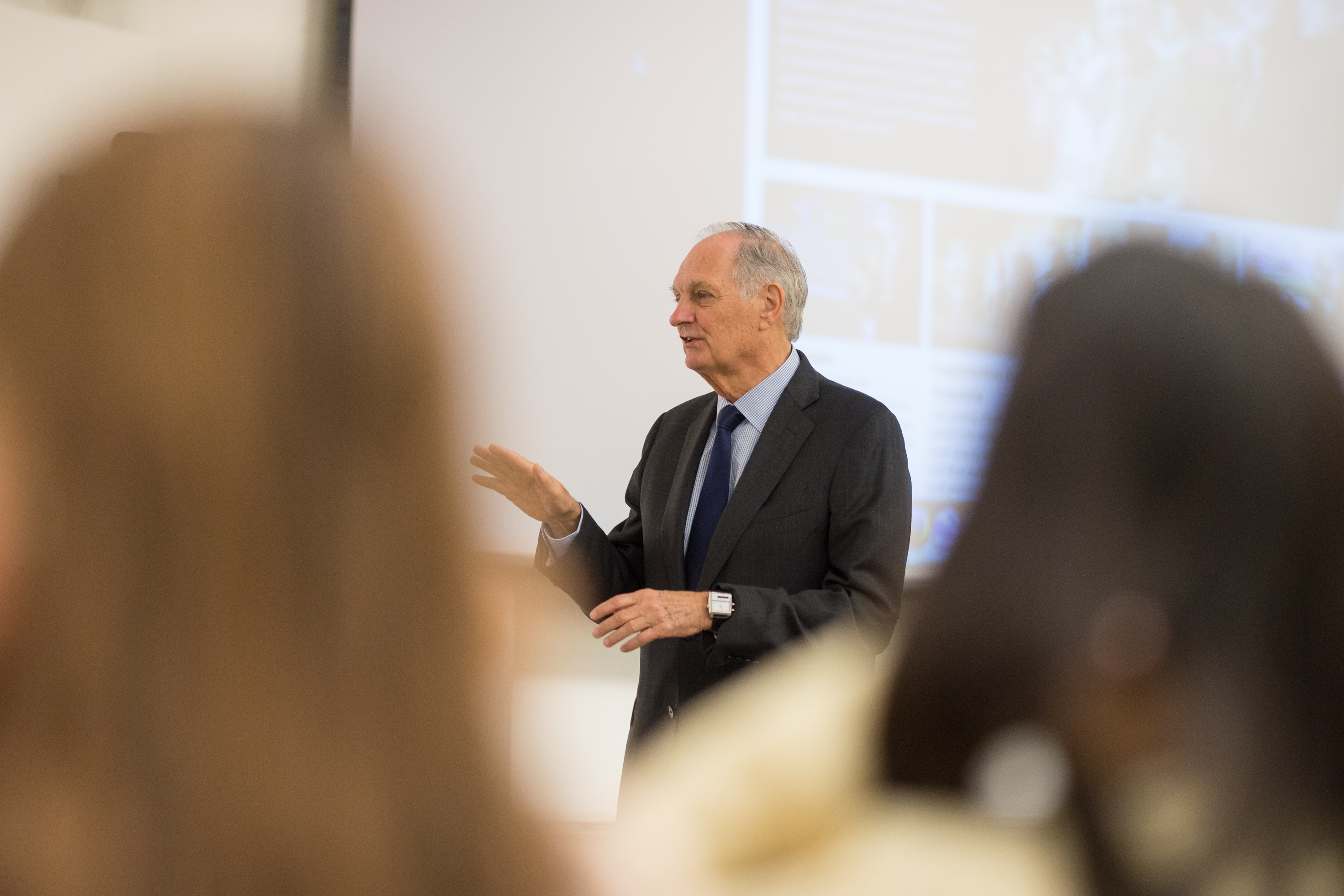In the image, an older man, who resembles either Alan Alda or Robert Alda, is captured mid-gesture while speaking at a seminar. He is positioned at the center of the frame, slightly turned in profile to the left, making his precise identity hard to determine. The man is dressed sharply in a gray suit paired with a blue tie and a white dress shirt. A square watch adorns his wrist, and his hands are animated as he speaks, with his right hand raised and his left slightly lower.

The background features a large projection screen displaying unclear images and text, set against a beige wall towards the upper left of the image. In the foreground, out-of-focus heads of two female attendees can be seen, framing the sides of the picture. The attendee on the left has red or light brown hair, while the one on the right has dark brown or black hair. The scene suggests an engaging lecture, possibly related to acting, given the context of the seminar.